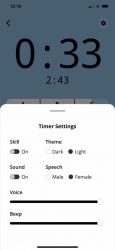The image depicts a slightly blurry interface of an electronic device or application. At the top, there is a large, dark blue box displaying "12-12-12" with an arrow pointing to the left and a small black sun icon on the right side. Below this, there are numerical values "0-33" and "2-43." The bottom part of the image is cut off, but three gray buttons with arrows are visible. A thin light gray line separates these elements from the white background below. 

The text on the white background appears to be settings for a timer. The first setting is partially obscured but includes the characters "S" and "B." Another setting is labeled "Dark and Light," with the "Light" option checked. Below this, a "Sound" setting is marked "On." Further down, there is a "Speech" setting with male and female options; the female option is selected. There is a thick black line, followed by settings labeled "Voice," "Deep," and additional black lines.